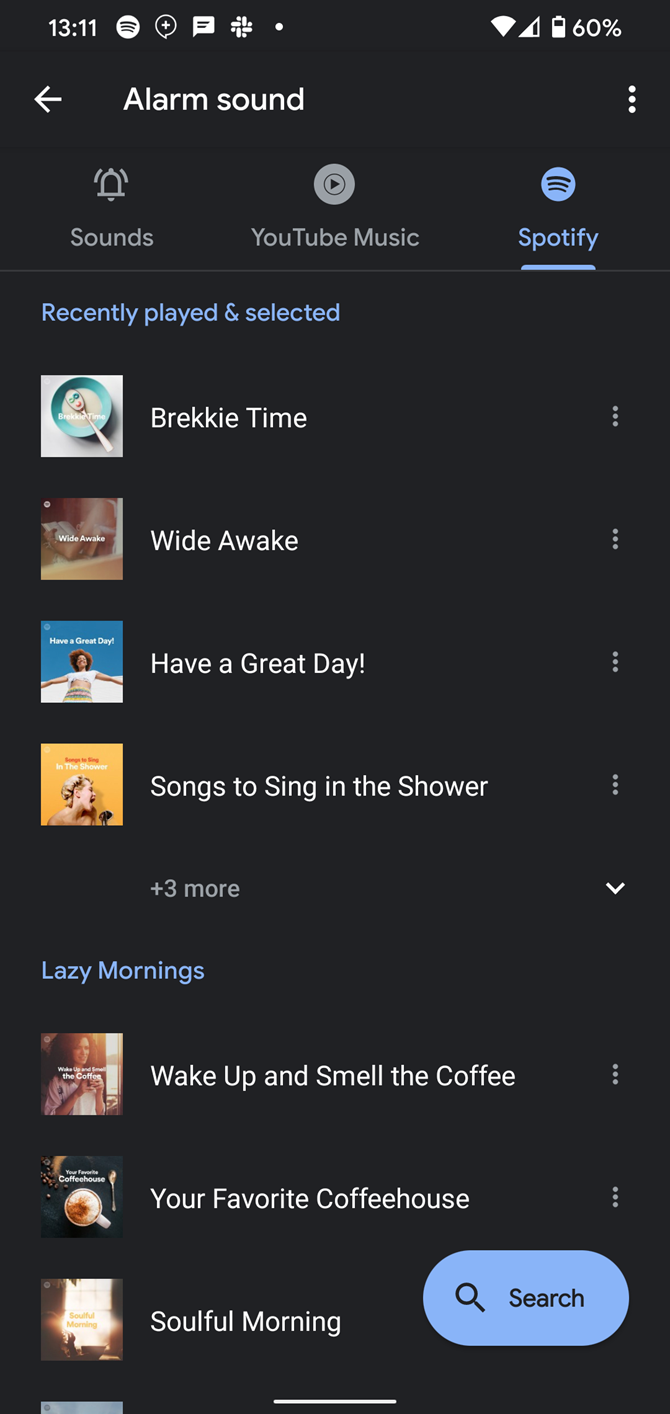The image displays a smartphone screen with various on-screen elements and icons. In the upper left corner, the time is shown as "13:11,” with icons for messages and other notifications nearby. On the upper right, there are signal strength bars for cellular and Wi-Fi data, and the battery level is indicated at 60%. Below, there is a navigation bar which includes a left-pointing arrow labeled "Alarm Sound" on the left side, and three vertically stacked dots (indicating a menu) on the right.

Further down, there are three tabs labeled "Sound," "YouTube Music," and "Spotify." The "Spotify" tab is selected, as highlighted by its blue color, while the other two tabs remain gray. A blue line beneath "Spotify" reinforces this selection. The next section is titled "Recently Played," also highlighted in blue. This section lists a series of songs or playlists, each accompanied by what appears to be an album cover icon. The listed items include:

1. "Breaky Time"
2. "Wide Awake"
3. "Have a Great Day"
4. "Songs to Sing in the Shower"

There is additional text indicating “plus three more” below these items, accompanied by a pull-down menu. 

Further down, a highlighted blue text reads “Lazy Mornings,” under which three playlists are listed, each with corresponding icons:
1. "Wake Up and Smell the Coffee"
2. "Your Favorite Coffee House"
3. "Soulful Morning"

In the bottom right corner, there is a light blue button with a black magnifying glass icon and the word "Search." The bottom of the screen features a white navigation bar centrally placed on a predominantly black background, with white fonts used for most of the text elements.